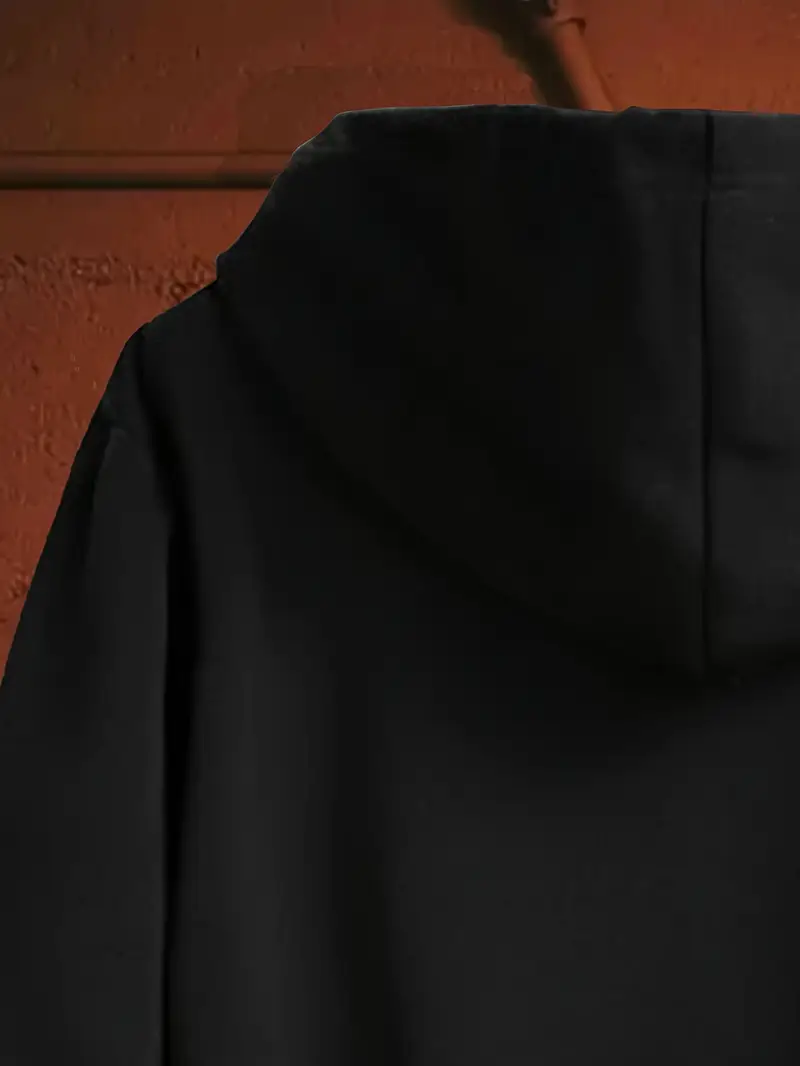This photograph showcases the back portion of a black hoodie, partially visible against a vivid red wall. The hoodie features a prominently stitched vertical seam running down the center of its hood. The wall behind the garment is painted red and adorned with metallic pipes, also red. One pipe runs horizontally across the image, while another pipe extends vertically in a slightly diagonal direction. The composition of the image is in portrait orientation.